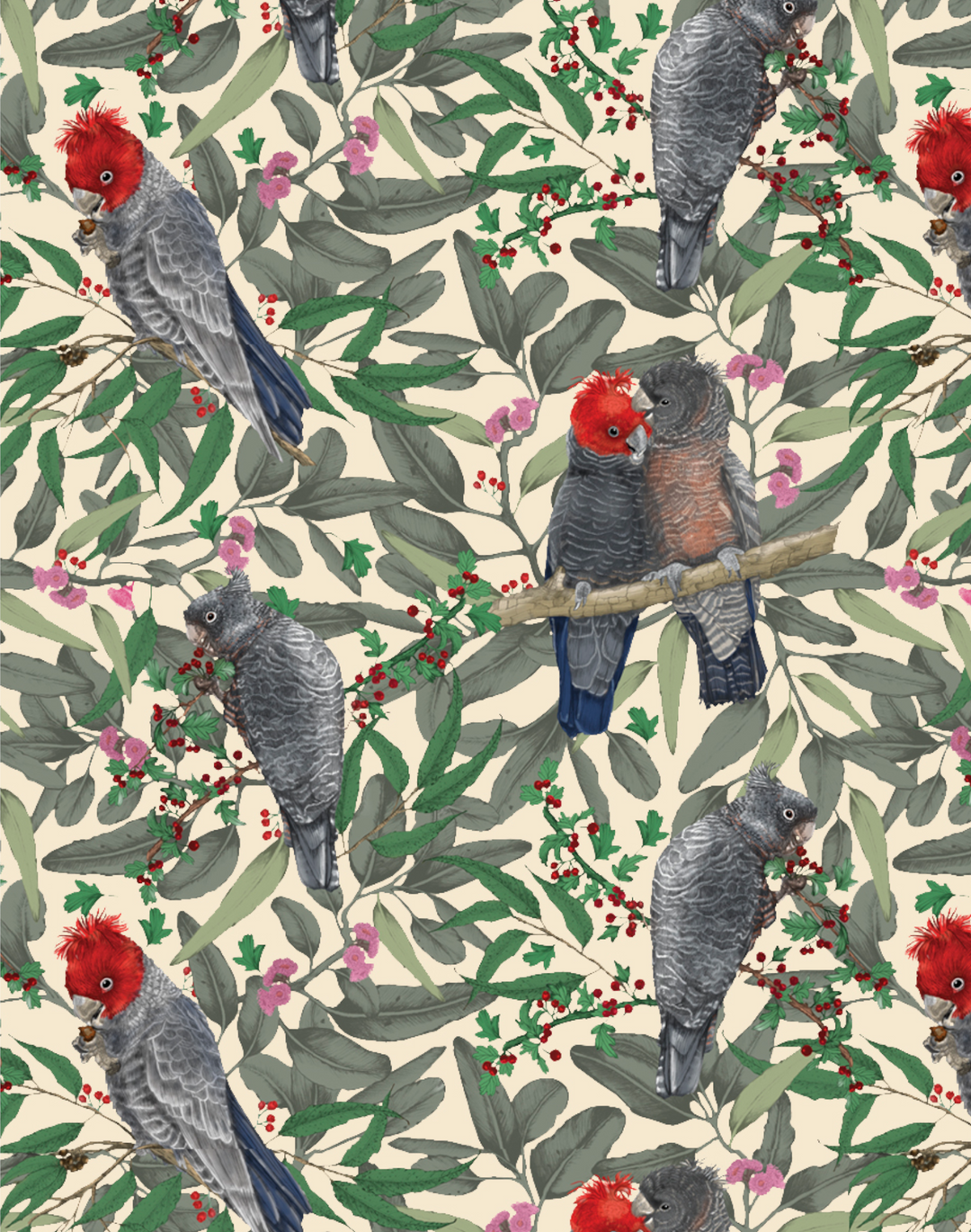The image is a detailed illustration of various parakeets set against a background of intricately drawn green leaves in differing shades. The artwork features several parakeets with distinctive red heads and gray bodies, accented by striking dark blue wingtips. Among them is a closely snuggling parakeet couple in the center of the image, one with a red head and gray body, and the other with a light pink body and gray head, both perched on a branch. Scattered leaves are interspersed with vibrant red berries and delicate pink and lilac flowers. The birds and foliage are carefully arranged on a beige to whitish-beige backdrop, giving the artwork a wallpaper-like appearance. The composition is vertically oriented, and some of the birds are cut off at the edges, adding a sense of depth to the scene.